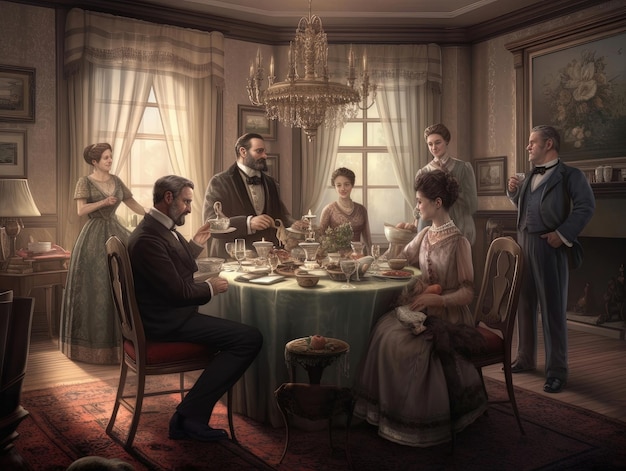The image, presumably a painting from the early 1900s or late 1800s, portrays a dimly lit, grand indoor setting featuring a round dining table adorned with a mint green tablecloth at the center. The muted colors and style of clothing contribute to an old-fashioned ambiance. The wooden floor is partly covered by a red rug, and a chandelier hangs from the ceiling. 

Seated at the table are four individuals: on the left, a man in a suit holding a cup and saucer looks towards a woman on the right, who has one hand on her lap and the other obscured behind the table. On the right side, a second woman sits, facing left, and another man, partially visible from behind her, completes the seated group. Standing in the room are five more people: to the far right, a man in a dark gray or blue suit with a black bow tie, next to him a very tall woman, then another woman who could be sitting or is very short, situated directly beneath the overhead chandelier. To her left stands a bearded man in a suit with a bow tie, followed by a woman in a long dark green dress with gold or tan details at the far left. The room features two large windows with open curtains behind the table and a large painting on the wall above the fireplace on the right-hand side.